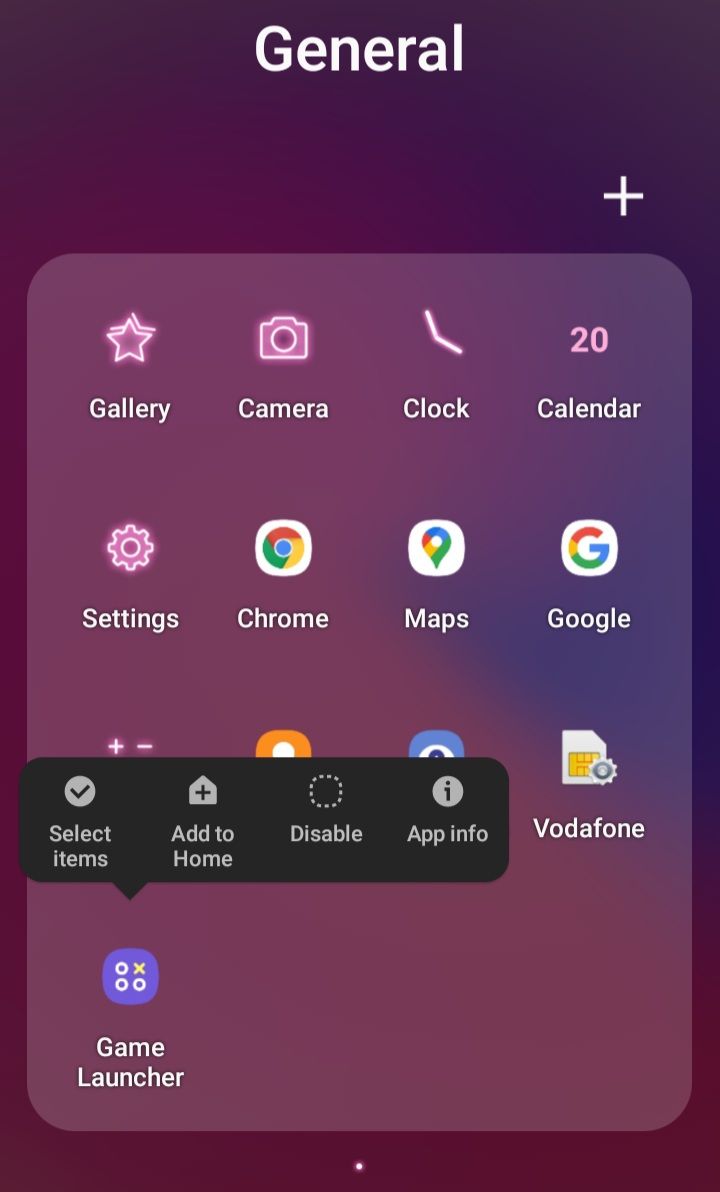This image depicts a screenshot taken from a mobile phone, specifically showcasing an app screen displayed under the "General" category. In the top section of the screen, the title "General" is prominently visible. Positioned at the lower right corner, beneath the title, there is a plus sign icon, indicating the possibility of adding more apps or icons to this category.

The screenshot includes a series of app icons: the first is "Gallery," followed by "Camera," "Clock," "Calendar," "Settings," "Chrome," "Maps," "Google," and "Vodafone." However, three other app icons remain obscured by an overlay pop-up screen.

This pop-up screen pertains to the "Game Launcher" app, revealing various settings and additional options for it. It presents four selectable options: "Select Items," "Add to Home," "Disable," and "App Info." The entire screenshot maintains a rectangular shape, offering a clear and organized view of the mobile interface and the functions available within the "Game Launcher" app.